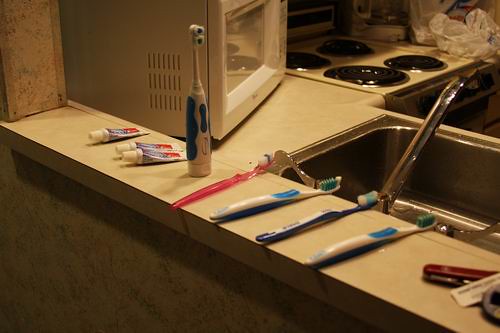The image depicts a kitchen countertop cluttered with personal hygiene items. Five toothbrushes are lined up on the countertop: three blue toothbrushes laying flat next to each other on the right, followed by a pink toothbrush to their left. An electric toothbrush with a white body and blue accents stands upright further to the left. Adjacent to the electric toothbrush are three small tubes of toothpaste, characterized by their white caps and red and blue bodies. Behind the countertop is a silver steel sink with a spout arching over it. Further in the background, there is a stove with four black burners and a white microwave with a glass window situated to the left. The design of the kitchen appears outdated, with noticeable scuff marks and an overall worn look.